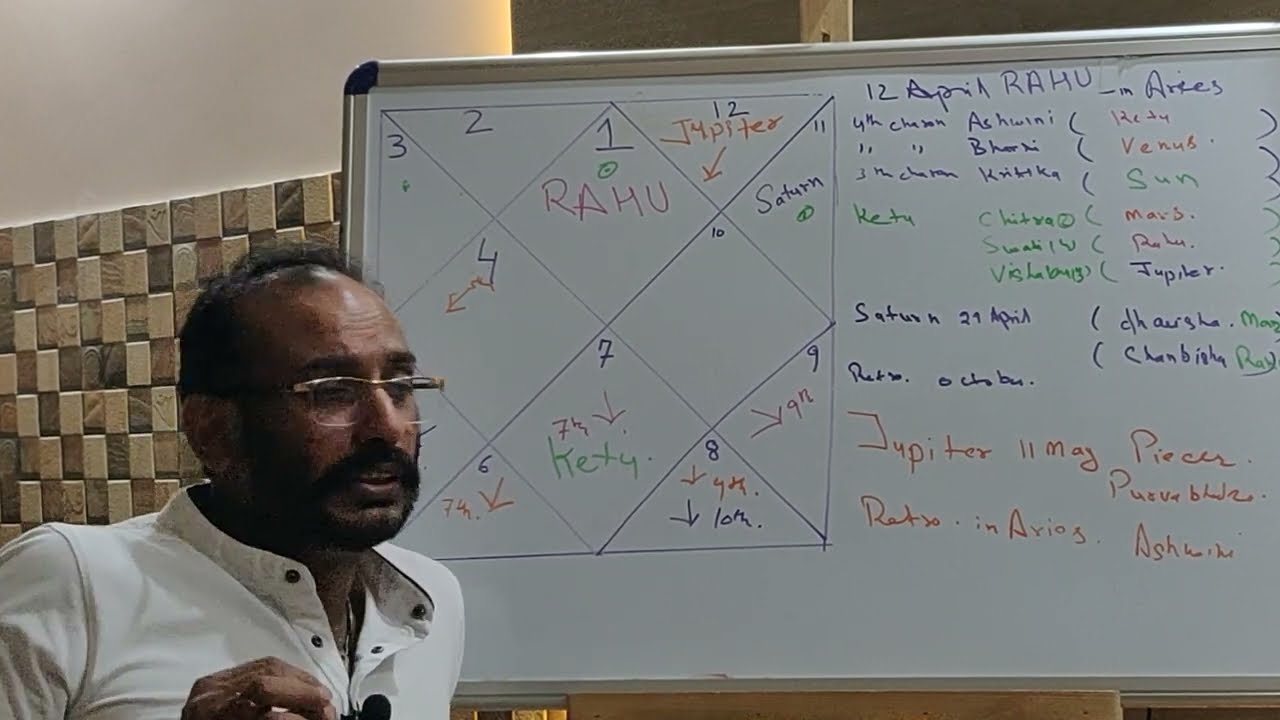The photograph captures an Indian man with dark skin and glasses, clad in a white shirt and sporting a thick mustache. He is actively teaching in an indoor setting, with his gaze directed towards a whiteboard on his right. The whiteboard is filled with diagrams and texts related to astrology, featuring names of celestial bodies such as Jupiter, Mars, the Sun, and Venus, as well as terms like Rahu and Ketu. Specific dates such as "12 April," "29 April," and "9 May" also appear alongside astrological signs like Aries. The background reveals a textured wall with various shades of brown tiles below a cream-colored section. The man’s hair is black and somewhat receding, and he's seen speaking, likely explaining the complexities charted out on the whiteboard.